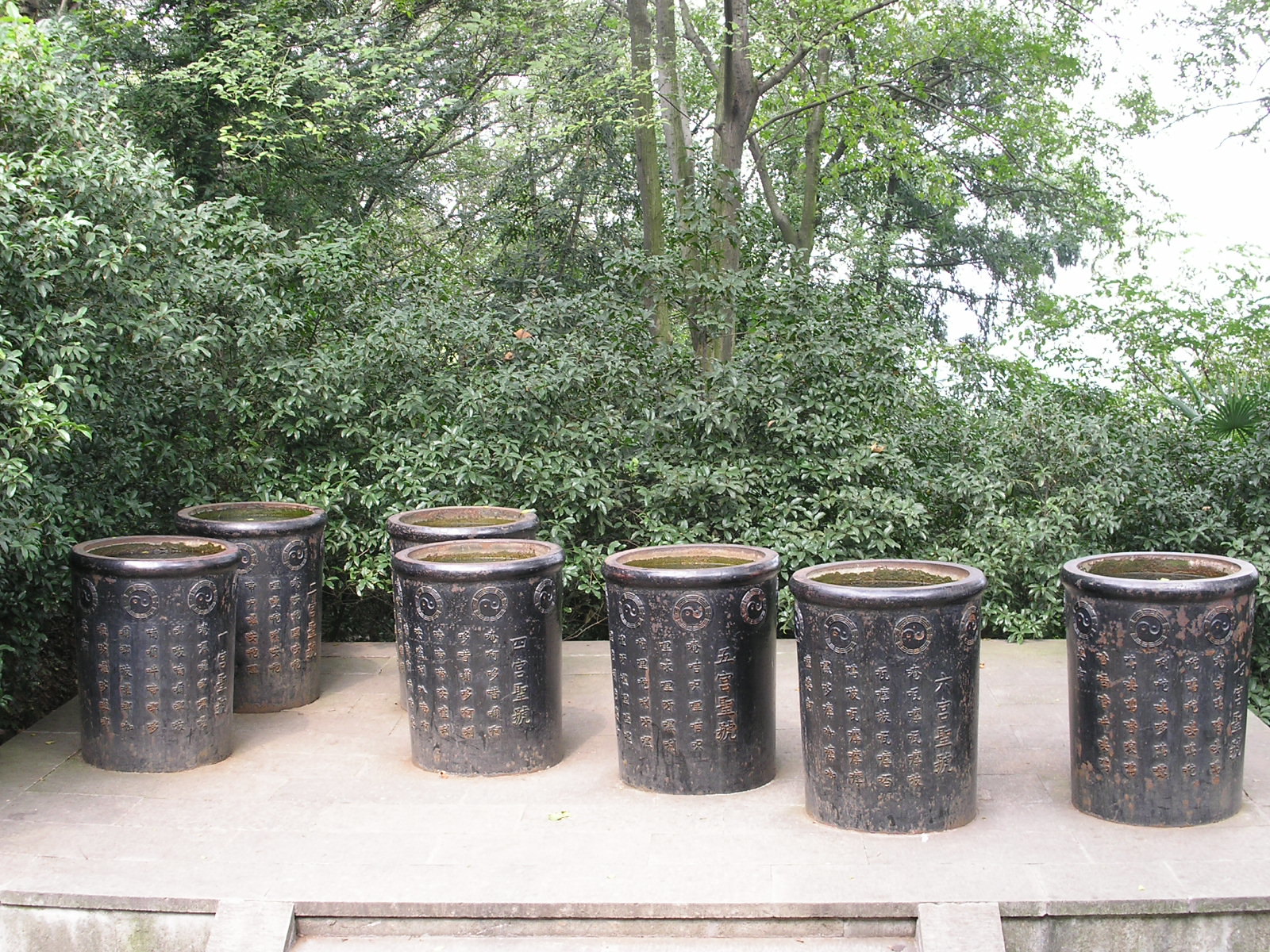The color photograph, taken outside on a bright sunny day, features a gray and white concrete platform set in front of a lush, green wooded area. On this platform are seven large, cylindrical metal pots, arranged in a neat row. These pots stand approximately a couple of feet tall and are predominantly black with a weathered, rusty dark brown or gray appearance, showing noticeable wear and scratches at their bases.

Each pot is adorned with intricate engravings, including multiple lines and rows of what appear to be Chinese symbols, and a series of yin-yang motifs circling their tops. The surface of these pots catches the sunlight, creating shining highlights, especially on their cylindrical tops.

Inside the pots, it is difficult to discern their exact contents; some suggest a greenish liquid or powder, while others speculate soil or even water. The sun, positioned behind the trees to the top right, casts a bright white light across the scene, illuminating the green leaves and large branches of the trees in the background. The sky appears almost pure white, providing a stark contrast to the vivid greens and the dark, weathered pots in sharp focus.